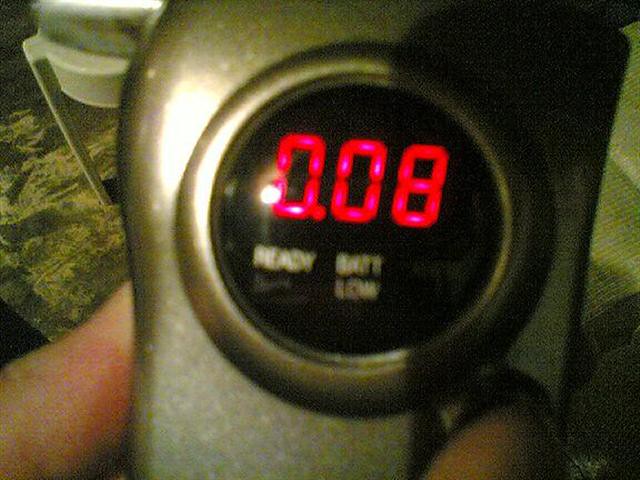The image depicts a close-up of a device that appears to be a stopwatch or a digital watch. The device features large red LED numbers displaying "0.08" prominently. Below the numbers, there's a slightly blurred section displaying the word "READY," and adjacent to it is an indication of a low battery, labeled either as "BATTERY LOW" or abbreviated as "BATT LOW." The device casing seems to be made of brass metal.

In the foreground of the image, two arms are visible. One arm appears to have a rash. The background reveals a green rug with gold tones and a stackable plastic outdoor chair. The vivid red numbers on the device stand out clearly against the otherwise muted background elements.